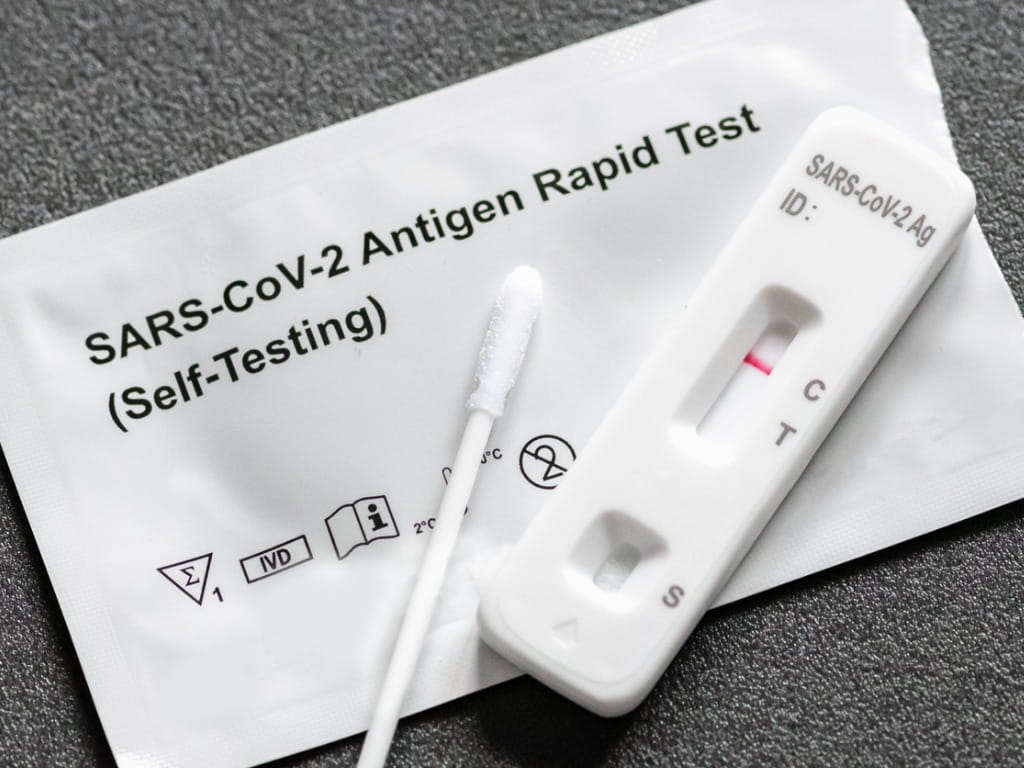The image depicts a COVID-19 test kit against a muted gray background, which appears to be either low-cut shag carpet or a textured tabletop. The main focus is the white plastic COVID-19 test wrapper that reads "SARS-CoV-2 Antigen Rapid Test (Self-testing)" in black text. Below this text, the wrapper features several symbols including an upside-down triangle with an "E" inside, a rectangle labeled "IBD," and an icon of an open book with a lowercase "i" on one of its pages. On top of the wrapper lies a swab, commonly known as a Q-tip, used for sample collection from the nose or mouth. The test kit's main testing device is white and rectangular, marked with "SARS-CoV-2 Ag ID" at the top. The device includes a testing strip area indicating "C" (control) and "T" (test), with a visible red line near the "C." This suggests the control line is active, indicating the test has been used. Additionally, there's an indentation marked "S" where the sample is placed. The overall color layout of the image transitions from lighter at the top to darker in the bottom right corner, adding depth to the scene.